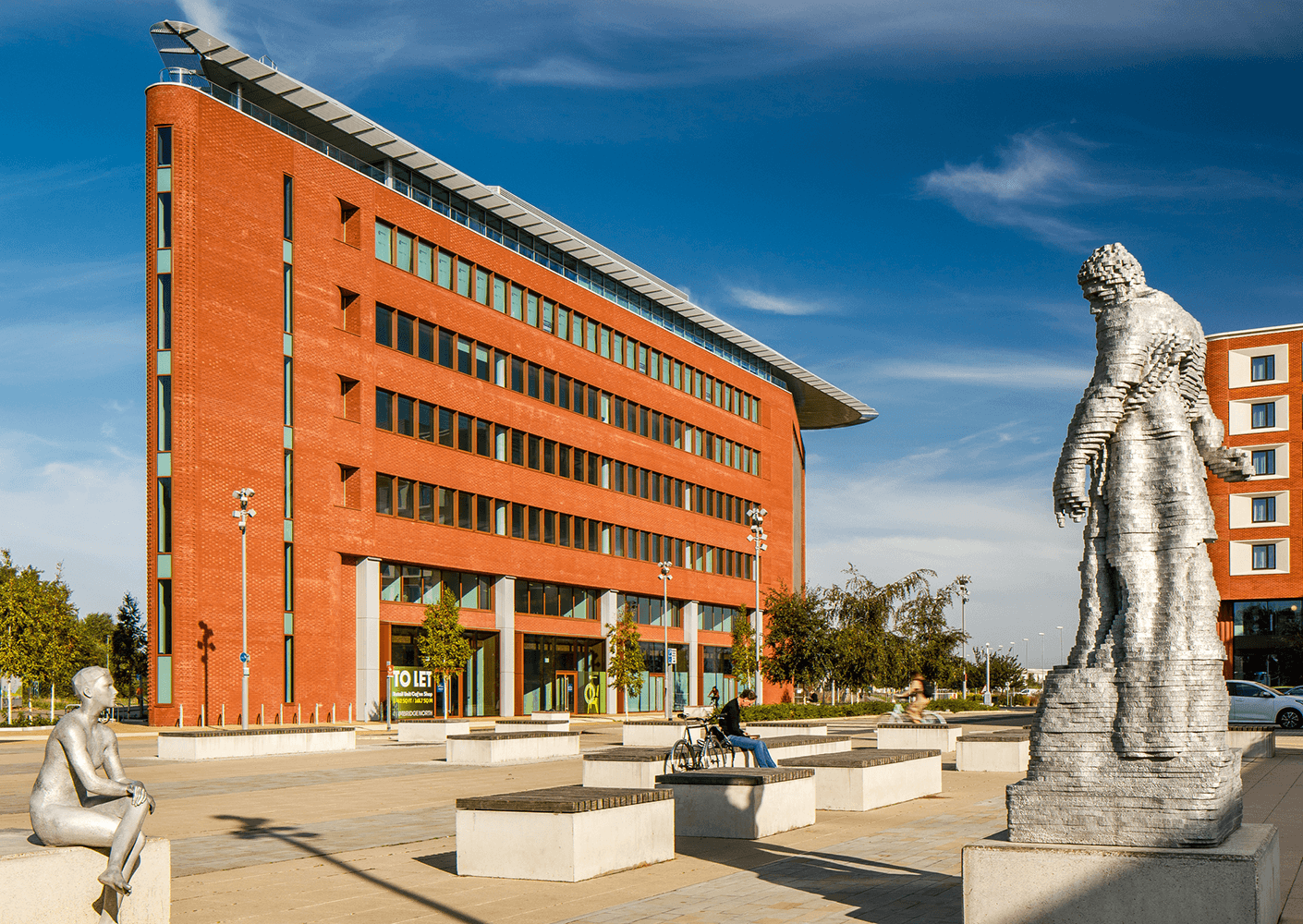The photograph captures a bright, clear day within a university quadrangle or a public square. The sky is a vivid blue with a few wispy clouds. The scene features a large hardscaped area filled with low concrete benches that provide seating throughout the space. 

Dominating the background is an unusual, six-story narrow brick building that tapers to a very slim edge on one side and widens out like a wedge. The building has an elongated surfboard-shaped roof, with long bands of brick alternating with rows of adjacent glass windows. A large sign out front suggests the building has rental spaces available.

In the foreground to the right stands a striking statue constructed from layers of stone or metal, resembling a tall male figure clad in armor or a robe, its contours crafted like a stack of misaligned nickels. On the lower left side lies another sculpture of a seated aluminum figure, with legs and arms crossed, gazing forward. 

A man is observed sitting on one of the concrete benches, a bicycle leaning against it. Surrounding him are additional sculptures and the scattered seating arrangements giving the area a gallery-like atmosphere. The whole scene is set against the backdrop of a clean, well-maintained city with some nearby trees.